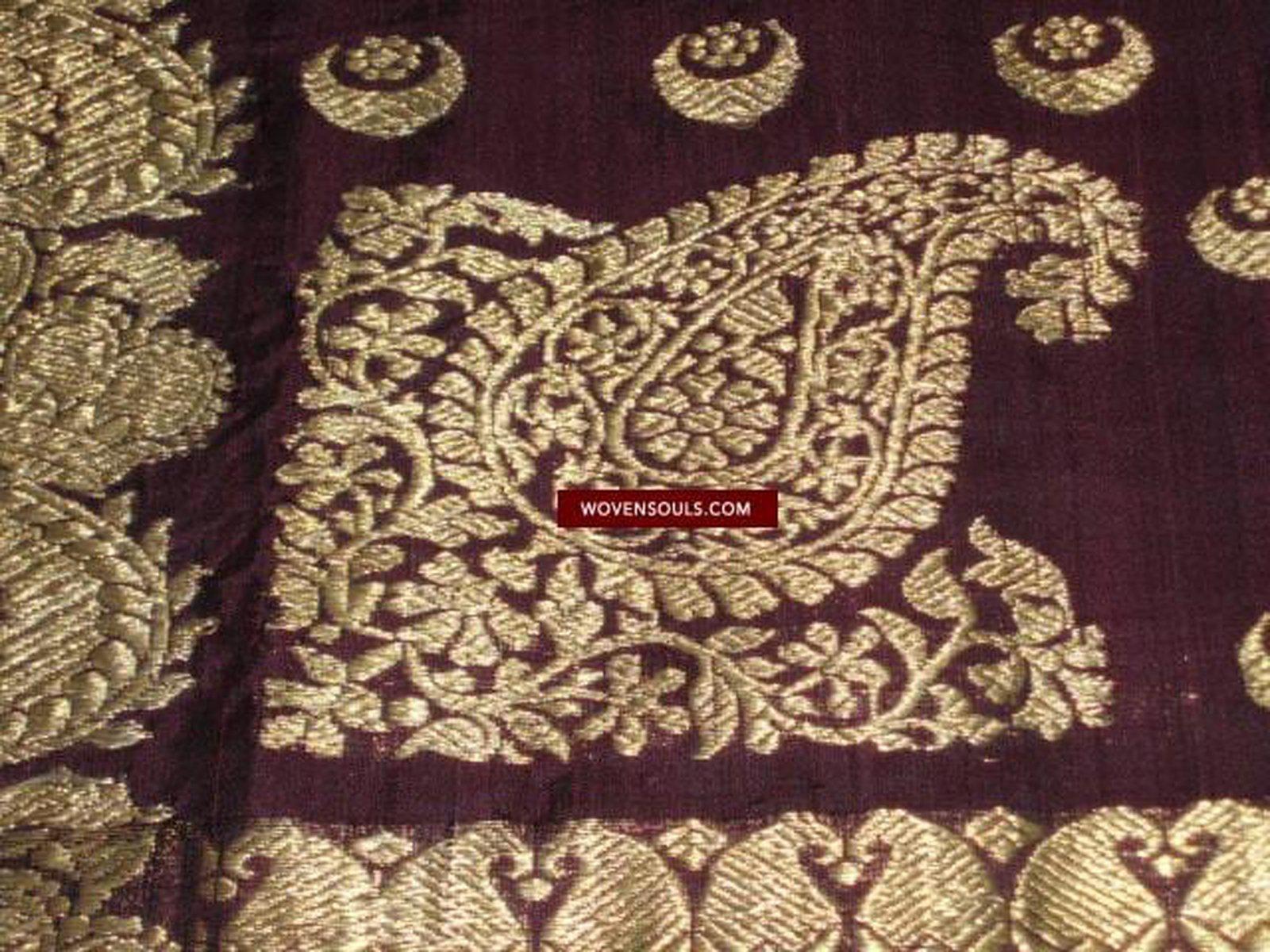This image is a close-up photograph of a woven fabric, perhaps a rug or tapestry, featuring a rich dark purple and gold color scheme. At the center of the image, a red square with white text prominently displays "WovenSouls.com." The background of the fabric is a deep purple decorated with ornate gold embroidery. Along the bottom and the left-hand side, there is a bright gold threaded border with intricate wave and sunburst patterns. The top edge showcases three gold, cornucopia-like designs. Centrally located is an ornate, pear-shaped gold pattern featuring intricate vines, floral elements, and curls. Additionally, along the right side near the top, there are small half-moon shapes with detailed decorations. The craftsmanship and intricate designs create a visually striking and detailed composition.